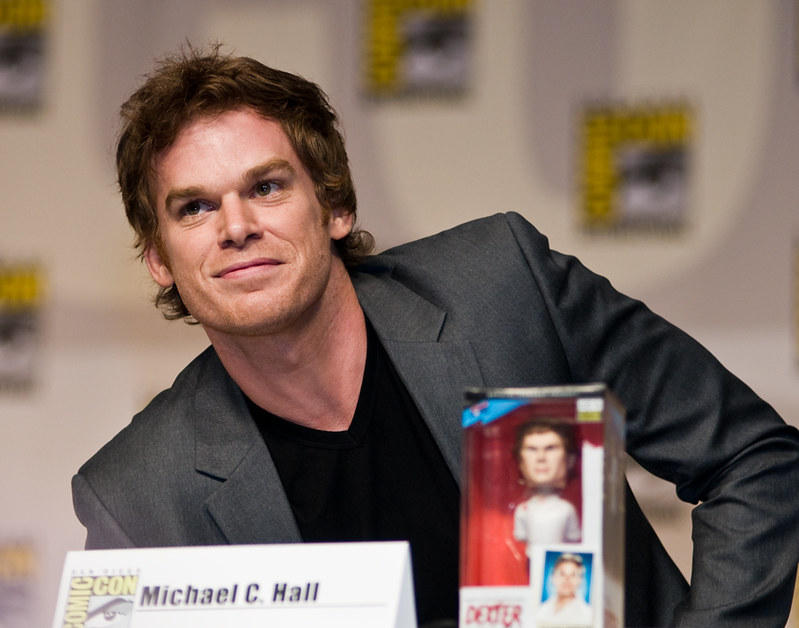In this image, the setting is a convention, likely Comic-Con, taking place indoors during the day. The background is blurry, making it difficult to distinguish details, but there appears to be an icon, possibly on wallpaper. In the foreground, a name tag prominently displays the text "Comic-Con, Michael C. Hall." Beside the name tag, there is a toy labeled "Dexter." At the center of the image sits a man, presumably Michael C. Hall, looking in the direction of the camera. The color palette of the scene includes black, white, yellow, light blue, red, gray, and tan. The man, name tag, and toy are the focal points, capturing the essence of a bustling, fan-filled convention atmosphere.